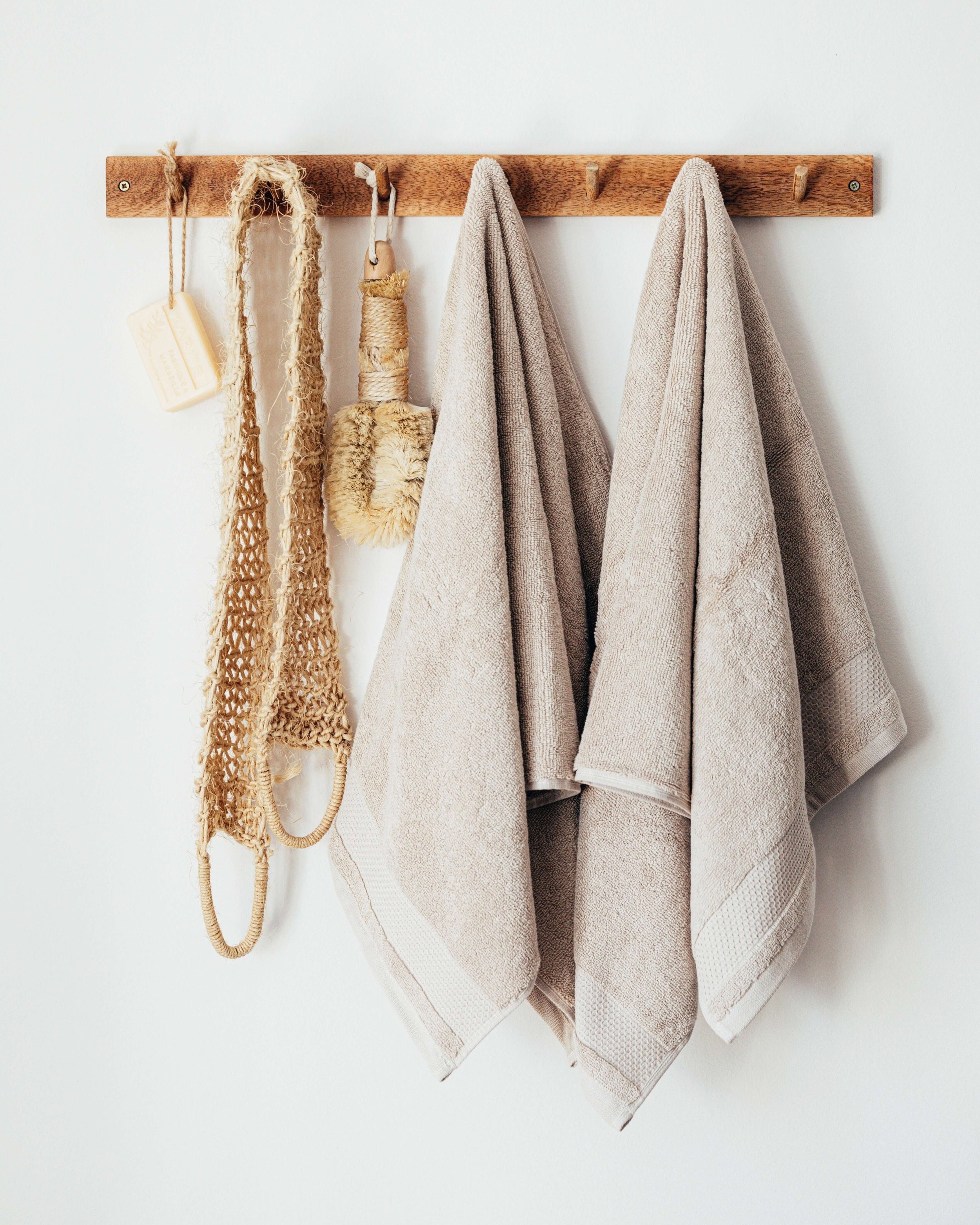The photograph depicts a minimalist wooden rack mounted on a pristine white wall. The rack is fastened with screws and features several pegs, from which various items are hung. From left to right, the first peg holds a bar of soap threaded with twine, possibly with a design etched into it. Next, a woven strap or scarf is elegantly draped, ending in loops of string. Moving further, a wooden dry brush with a twine handle hangs from another peg. Adjacent to it, a beige or brown towel is suspended, followed by an empty peg. The subsequent peg holds an identical towel in the same earthy hue, and the last peg on the far right remains empty. The overall composition is clean, simple, and showcases the utilitarian beauty of the arranged items.